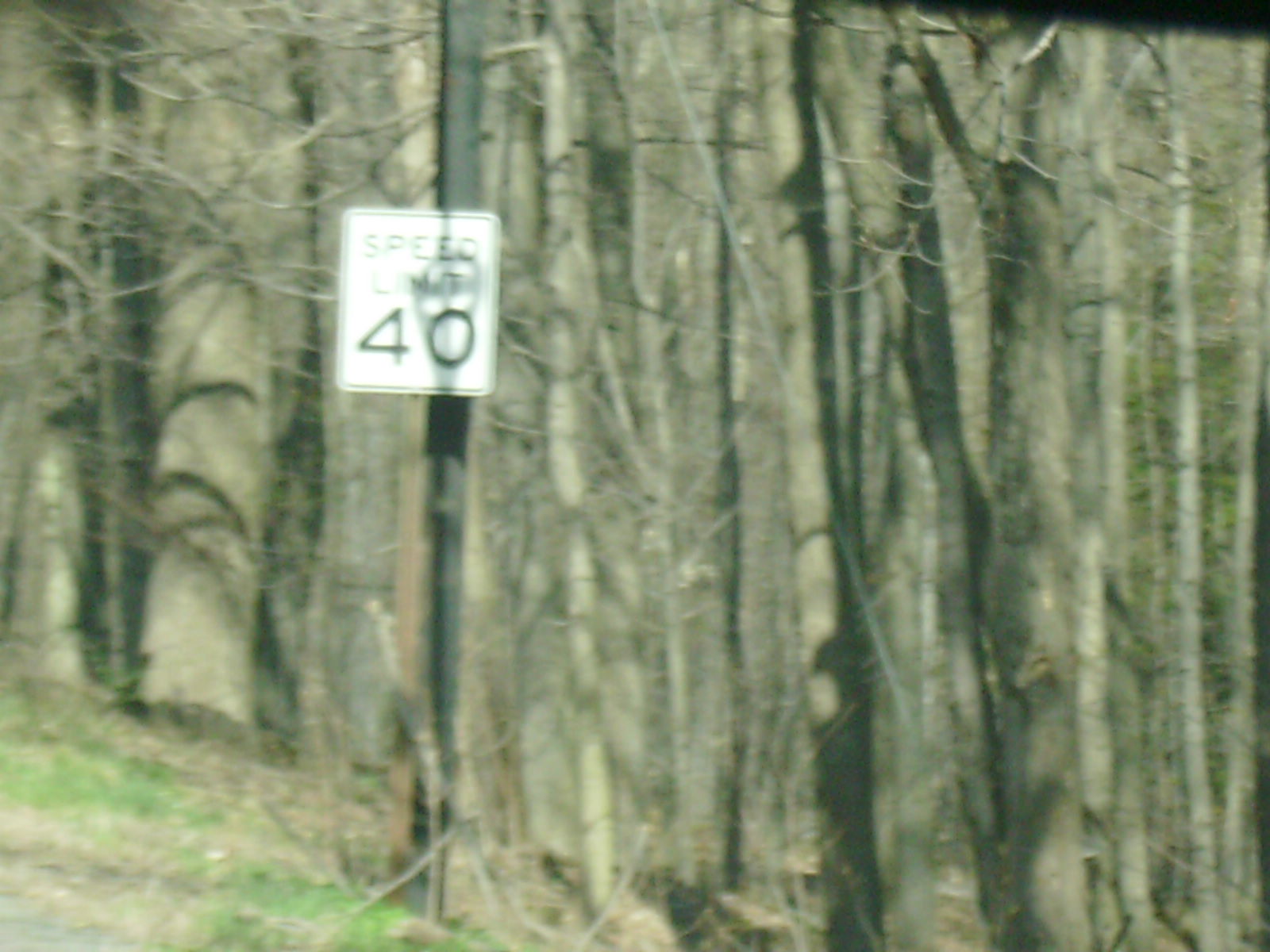This image is a highly blurry photograph likely taken while someone was driving. Dominating the scene is a white speed limit sign with black lettering that reads "Speed Limit 40," affixed midway up a black pole. A circular shadow with a cross, possibly either a shadow or graffiti, partially obscures the '0' in "40." The setting is outdoors on a bright, sunny day. In the background, there are numerous trees, most of which are bare, suggesting a winter or late autumn timeframe. A few trees on the right side display some greenish-yellow foliage. The ground below features patches of dirt with some green grass. The image's overall blurriness impedes clear details, with a black corner visible in the upper right hinting it might have been taken through a car window or from a screen. Additionally, there's a single metal line extending from the pole diagonally towards the bottom right, cutting off due to the blurriness. A small section of the road is visible in the bottom left corner of the frame.